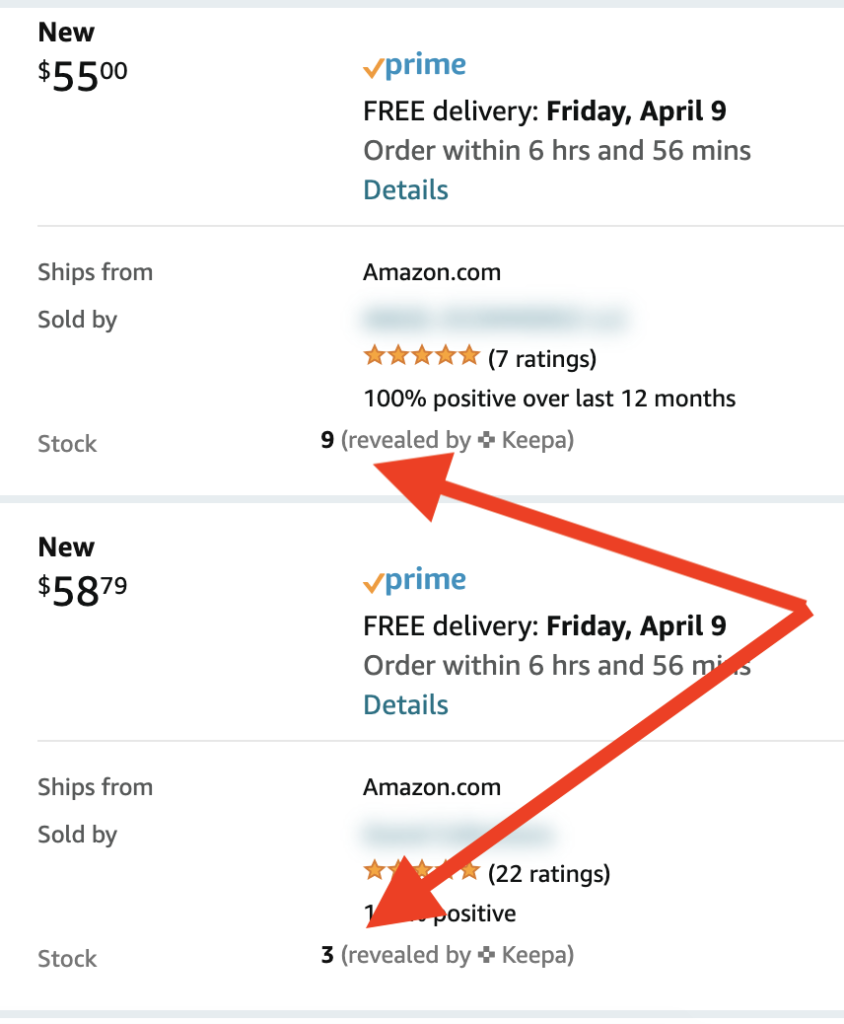The image is a vertical screenshot showcasing detailed information about two items listed on Amazon. The background is entirely white, framed at the top and bottom by thin gray horizontal bars. At the top, it's noted that the items ship from Amazon.com and the seller's name is obscured by a gray blur. The first item boasts a perfect five-star rating from seven reviews, maintaining 100% positive feedback over the past seven months. Inventory details, uncovered by the tool Keepa, reveal that only nine units are available. The second item, listed at $58.79 with Amazon Prime eligibility, assures free delivery by Friday, April 9, provided the order is placed within six hours and 56 minutes of viewing. Similar to the first item, it ships from Amazon.com with the seller's name blurred out. This product also has a five-star rating from 22 reviews, holding a 100% positive feedback score, with only three units in stock according to Keepa. Two red arrows on the image, connected at their bases, point towards the sections that mention "revealed by Keepa".